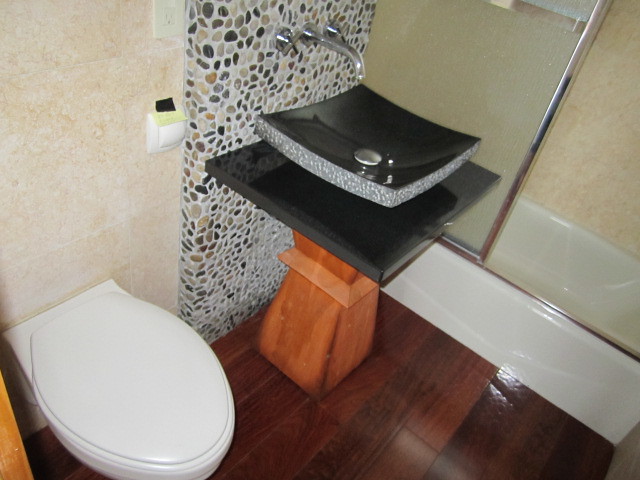This photograph captures the interior of a contemporary bathroom characterized by its modern design elements. The floor is laid with rich brown wooden planks, adding warmth to the space. In the lower left corner, a sleek white porcelain toilet, mounted directly to the beige and gold marble wall, lacks a conventional base, heightening its minimalist appeal. 

Adjacent to the toilet, a white square object is affixed to the wall, likely a flush panel or a decorative element. A section of the wall protrudes slightly, featuring a unique sea glass montage set in white concrete, serving as both an artistic accent and a partial room divider.

Dominating the foreground is an innovative sink design. The sink comprises a gracefully curved gray glass bowl adorned with subtle white and blue accents on its sides. Below the bowl, a matching gray glass rectangle enhances the modern aesthetic. The base of the sink is crafted from wood, providing a balanced contrast to the glass and marble textures. Completing the sophisticated look, the faucet and handles are mounted directly onto the wall, ensuring a clean and uncluttered appearance.